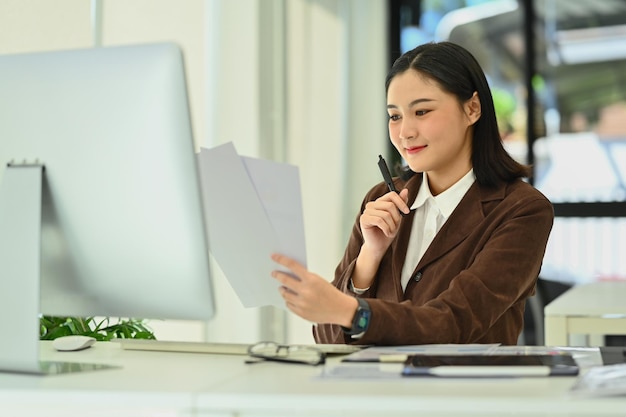This detailed photograph captures a scene of a woman seated at a modern white desk in what appears to be her office. The woman, who has dark brown hair, is dressed in a brown velvet button-down blazer layered over a white collared shirt. A watch adorns one of her wrists. She holds two pieces of paper in her right hand and a pen in her left, indicating she may be reviewing some documents. Her expression is pleasant, depicted by a slight smile as she focuses on the papers.

The desk is well-organized and includes an array of professional items: sheets of paper, digital devices, a pair of glasses, a computer mouse, and a computer monitor. The monitor, displayed prominently on a stand to her left, has its back and side somewhat out of focus but adds to the modern aesthetic of her workspace. 

The background is predominantly white, with a large open window allowing natural light to filter in, enhancing the crisp and clean atmosphere of the office. Greenery is subtly visible, and a plant can be seen on the floor behind her desk. Additionally, there is another white table behind her, further contributing to the minimalist design of the space. Elements like a clipboard or other indistinguishable items also populate her desk, reinforcing the businesslike setting. The overall lighting suggests it might be morning.